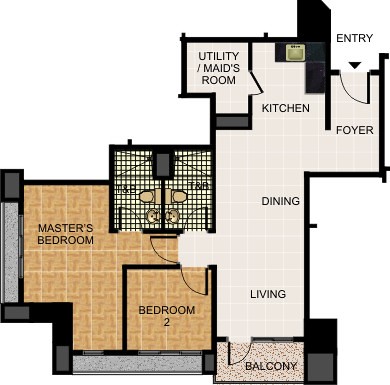This image is a top-down layout of a house. The entrance is located on the right side, leading into a small enclosed area where the wall extends slightly beyond the entryway. This area opens up into a foyer. 

From the foyer, there is a narrow turn that leads directly into the combined kitchen and dining room area. The kitchen is situated on the right with a sink on the upper side and an oven to the right. To the left side of the kitchen, there is a door that provides access to a utility or maid's room. 

Moving past the kitchen, the dining room seamlessly transitions into the living room, forming a large open space. This living area includes a door that opens out onto the balcony.

Approximately halfway through the living area, a left turn leads into a hallway. This hallway provides access to the master bedroom at the end. The second bedroom is located to the left off this hallway, while immediately to the right, there is a door leading to one bathroom. Further down the hallway and also on the right, there is another door to a second bathroom, with the bathrooms oriented in opposite directions.